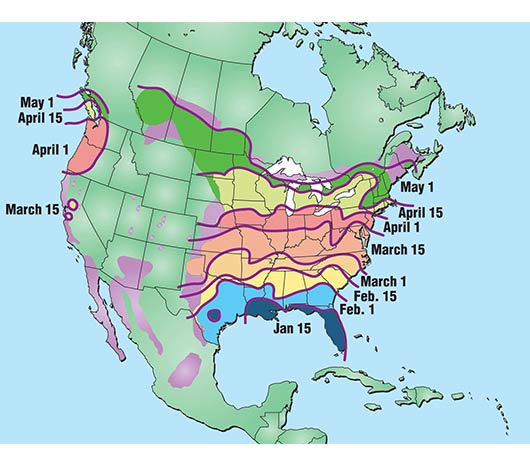This image is a detailed meteorological map of North America, vividly colored to represent various dates. The map shows North America, featuring green land masses surrounded by light blue ocean. Mexico is at the bottom, with Cuba and the Bahamas to the right, followed by the United States, and topped by Canadian provinces. The map is overlaid with irregularly shaped, color-coded zones indicating different dates, likely representing climate-related data.

Starting from the south, the state of Florida is filled in dark blue and labeled January 15th. Above it, a light blue area covers the southern half of Georgia, Alabama, Mississippi, the northern half of Louisiana, and the southern half of Texas, dated February 1st. Moving upward, a light yellow zone includes South Carolina, northern Georgia, northern Alabama, northern Mississippi, the southern part of Arkansas, and the middle part of Texas, marked February 15th. Above this is a light orange band labeled March 1st, followed by a darker orange area indicating March 15th.

A red-orange flow spans from New Jersey to Nebraska and is labeled April 1st. Further north, light green covers parts of Minnesota down to Iowa and extends across various states, marked April 15th. An olive green area indicates May 1st, flowing horizontally from the Eastern Seaboard to Canada. A purplish zone covers parts of Canada, New England, North Dakota, Minnesota, Wisconsin, and Michigan, labeled May 1st.

On the West Coast, a purple region runs down California, dated March 15th, with the red area on the coast of Washington and Oregon marked April 1st. Above this, in the Vancouver area, a yellow zone is labeled April 15th, with another yellow area above it marked May 1st. The color transitions and their flow-like, irregular borders suggest the progression of meteorological phenomena over time.